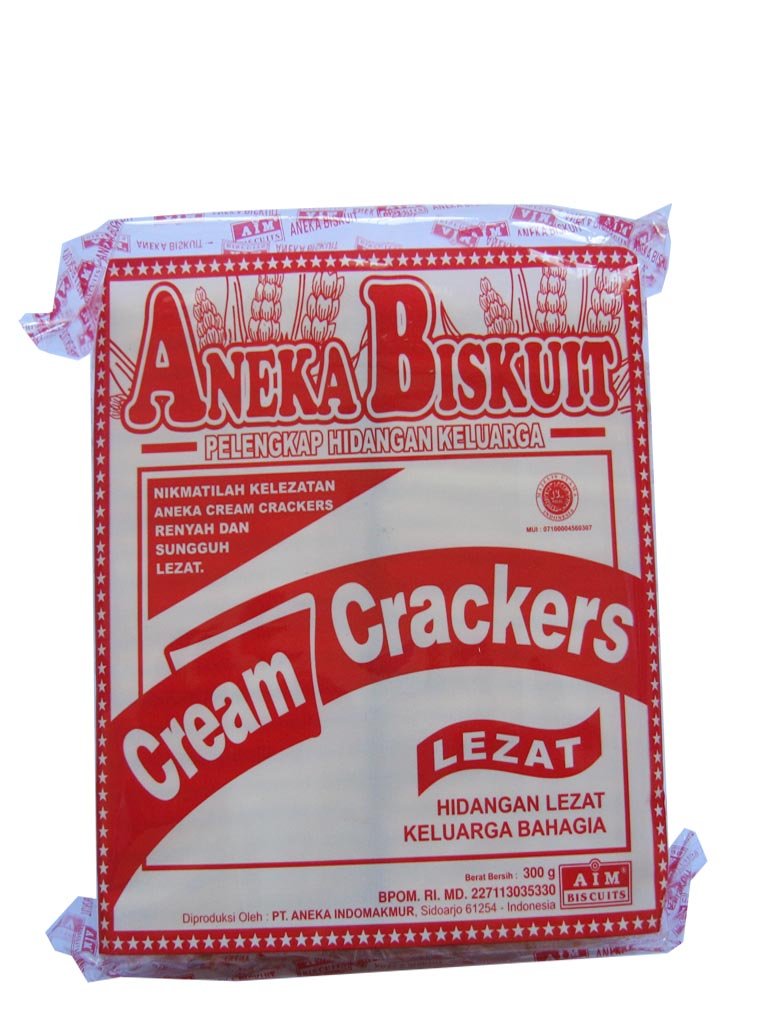The image depicts a shiny, cellophane-type plastic bag, sealed at the top and bottom, containing a package of crackers. The packaging is predominantly white with prominent red labeling. At the top, the text reads "Aneka Biskut" in red on a white background. Below this header, a red-outlined banner states "Pelengkap Hidangkan Keluarga." In the center of the package, a large banner in red font prominently displays "Cream Crackers." Below this central banner, there are more foreign language texts which include "Nikmatila Kelizatan Aneka Cream Crackers Renyah Dan Sungguh Lezat" and another banner stating "Lizat." In one corner, a square label mentions "AIM Biscuits," and along the bottom edge, there is a decorative red border adorned with white stars. The background of the main title area features an image of wheat, emphasizing the crackers' ingredients. The overall design suggests a pull-open type of package with clear seam lines at the top and bottom, indicating where it can be opened by hand.